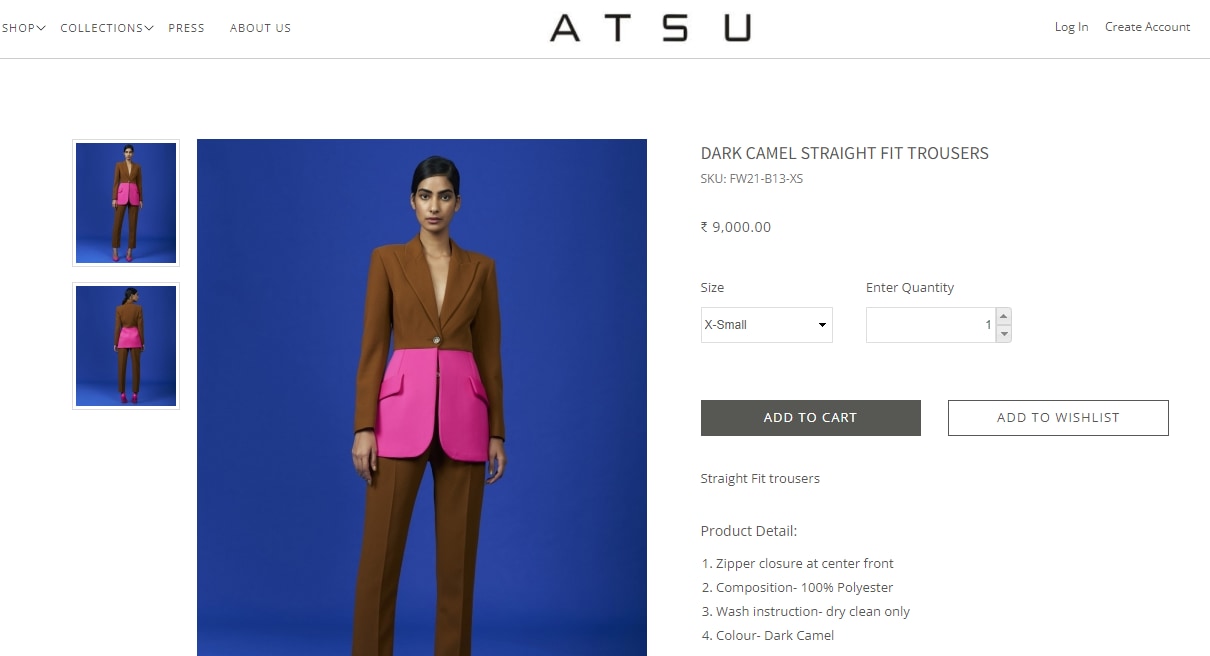This screenshot captures a computer screen displaying a retail website with its upper navigation bar prominently featuring the brand name "A T S U" in bold, black, capital letters, each letter separated by a space. On the far left of the navigation bar, the word "shop" appears in gray with a downward arrow indicating a drop-down menu. Following this are the options "collections" with another downward arrow, "press," and "about us." On the far right of the navigation bar, the options "login" and "create account" are displayed for user interaction.

The left-hand side of the screen features two rectangular images set against a vibrant royal blue background. Each image presents a model, likely of Indian descent, wearing a striking outfit consisting of a brown jacket with a hot pink lower half, buttoned centrally without an undershirt, and brown trousers. Her dark hair is styled back, and she faces the camera with her arms at her sides, exuding poise and confidence.

To the right of these smaller images is a larger, similar image of the same model in the same outfit and background, emphasizing the featured clothing item. Adjacent to this primary image, gray text reads "Dark Camel Straight-Fit Trousers" along with the item's price. The interface allows the user to select their size and quantity before choosing to add the item to their cart or their wish list through rectangular buttons, completing the shopping experience with ease. This well-organized layout combines visual appeal with user-friendly navigation.